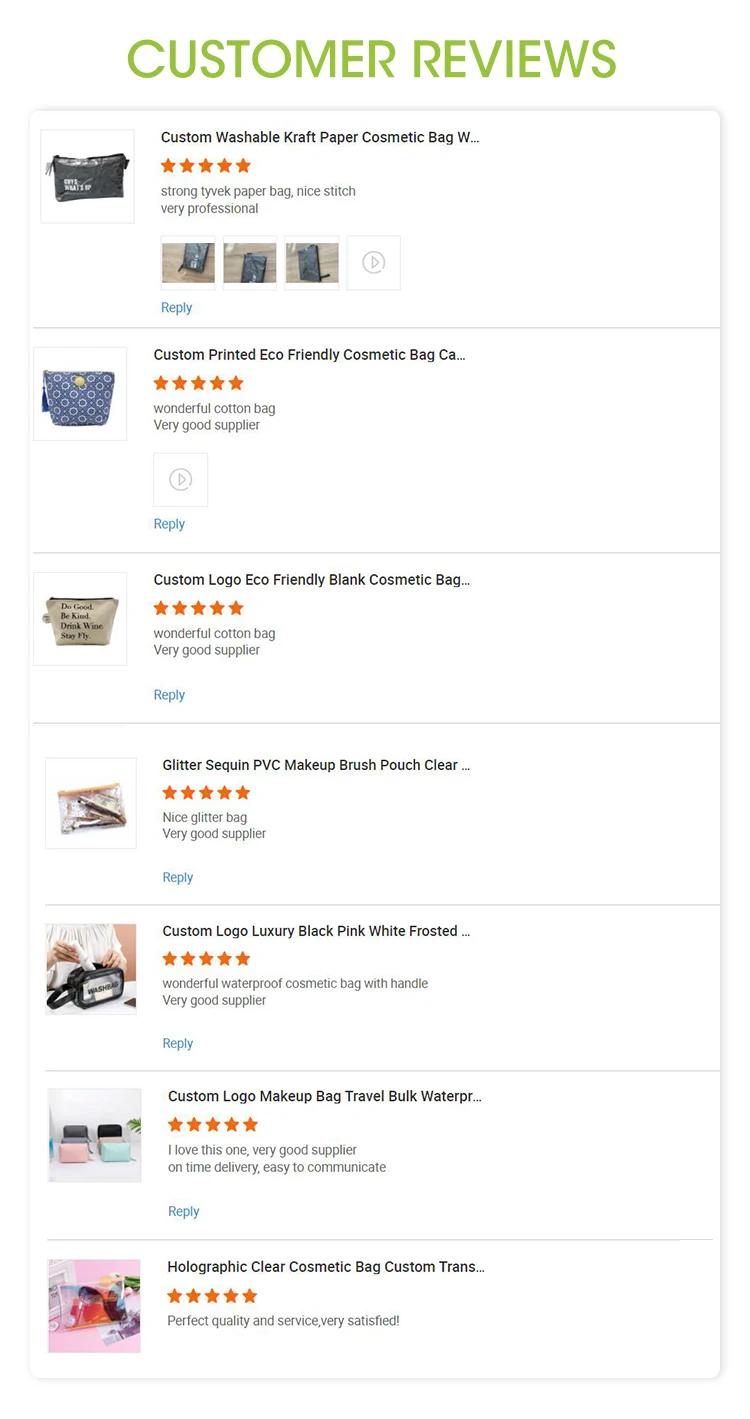Customer reviews for a custom washable craft paper cosmetic bag highlight its durability and eco-friendliness. A professional seller provides custom printed, eco-friendly cosmetic bags, garnering five-star ratings for the exceptional quality and prompt replies. One cosmetic bag features a sleek black design made from strong Tovic paper, perfect for nighttime use. Another review praises the product's luxury, describing a beautiful cosmetic bag adorned with glitter sequins and pivoting details, also receiving five orange stars. Additionally, a cosmetic bag boasts a white square with blue circles resembling a sun, showcasing the high-quality craftsmanship and attention to detail. Overall, customers are extremely satisfied with the product's customizability, quality, and the supplier's excellent service.